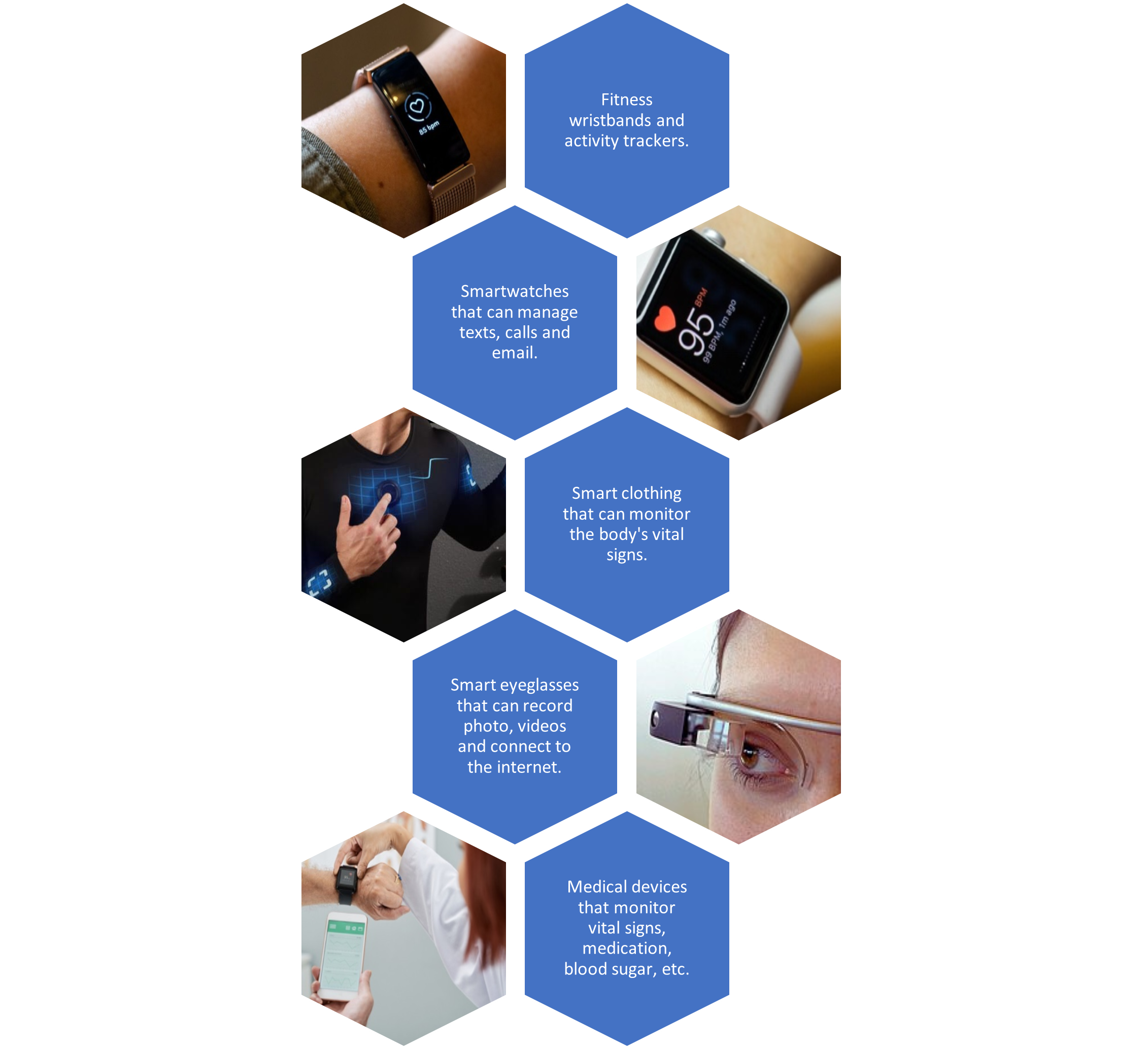This image, likely an advertisement or PowerPoint presentation slide, presents an infographic for smart devices on a white background. The composition includes a staggered tower of ten hexagons arranged in five rows, each row comprising an image hexagon and a text hexagon. The images depict various smart devices, while the text, in white font against a blue background, details their functionalities. Starting from the top left, the first image shows an arm wearing an activity tracker or fitness wristband, accompanied by text about fitness bands and activity trackers. Adjacent to that, a smart watch capable of managing texts, calls, and emails is showcased. The next row features smart clothing that monitors the body's vital signs, illustrated by a black shirt integrated with electronics. This is followed by an image of smart eyeglasses, such as Google Glass, which can record photos and videos and connect to the internet. The final row highlights medical devices that monitor vital signs, medication, and blood sugar, depicted with a doctor holding an arm equipped with a smartwatch and phone. The images and text together provide a comprehensive overview of various smart wearable technologies and their functionalities.